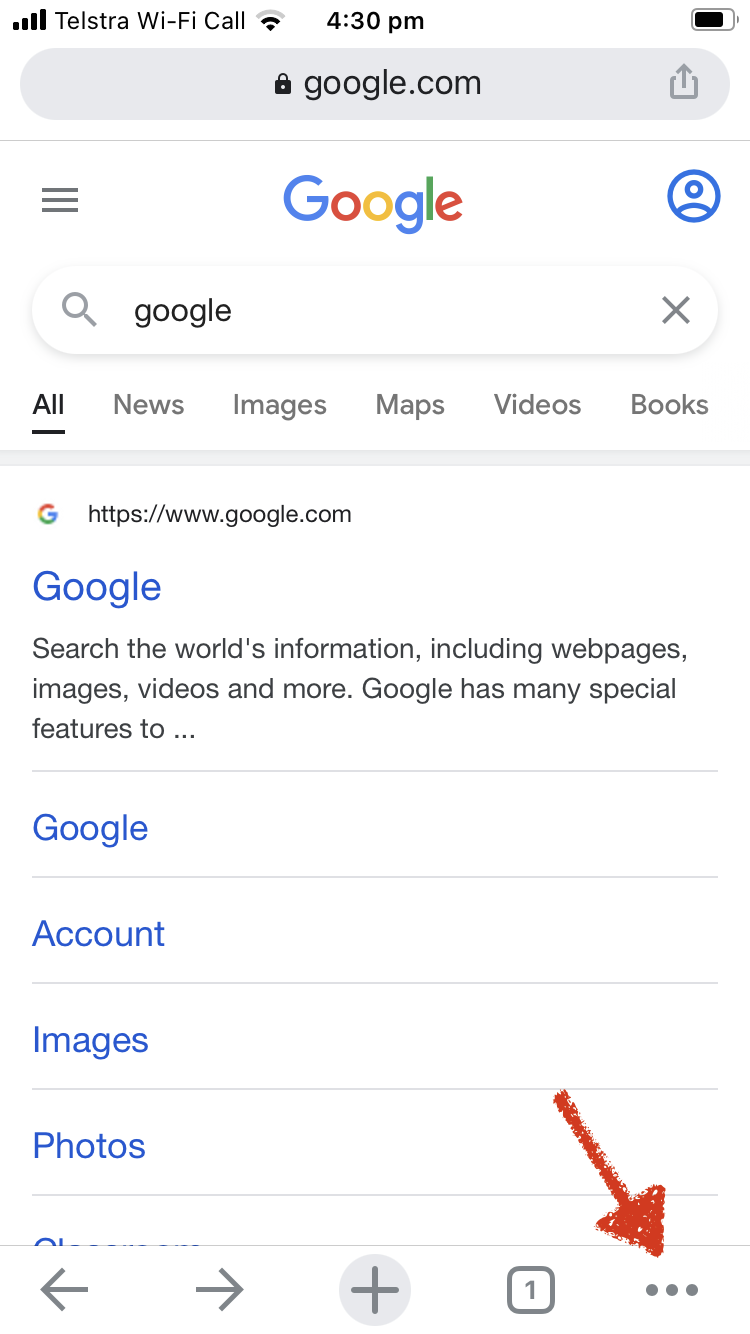The image is a screenshot from an iPhone, displaying the Safari browser. The user has navigated to google.com, as indicated in the URL bar at the top of the screen. In the Google search bar, the word "Google" is also typed in. The first search result is the official Google link, accompanied by a brief description: "Search the world's information, including webpages, images, videos, and more. Google has many special features to..." The description is cut off at this point. Below the primary link, there are navigational links labeled "Google," "Account," "Images," and "Photos." Towards the bottom of the screen, there is a red arrow drawn, pointing to the three dots located in the bottom right corner of the screen, indicating additional options or settings.